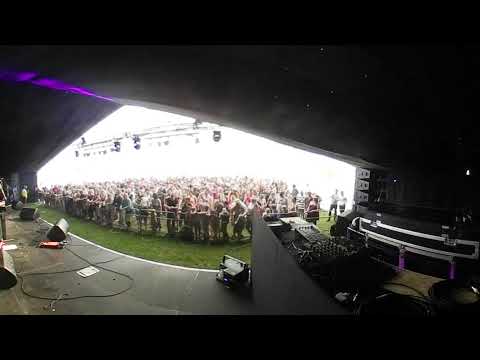The photograph captures an expansive concert arena from a unique perspective beneath a soundstage. The stage itself is covered and features a variety of sound equipment, including DJ pads and dials, large black amps with metal linings, cables arranged in curves, and hanging lights under the canopy. The stage is predominantly black and stretches from the center left of the image to the bottom right side, appearing larger due to a fisheye lens that adds a distorted, wide-angle effect. Purple lighting illuminates the top of the stage structure, contrasting with the overcast, white sky outside. In the foreground, a silver metal barrier separates the stage from an audience that extends over a patch of green grass. Hundreds of concert-goers stand behind this barrier, their figures minimized by the lens's effect. The overall atmosphere suggests a seamless blend of indoor and outdoor spaces as the open canopy allows a view of the expansive, grassy audience area. There are no visible performers on stage, save for an indistinguishable figure possibly located to the very left-hand middle of the stage.